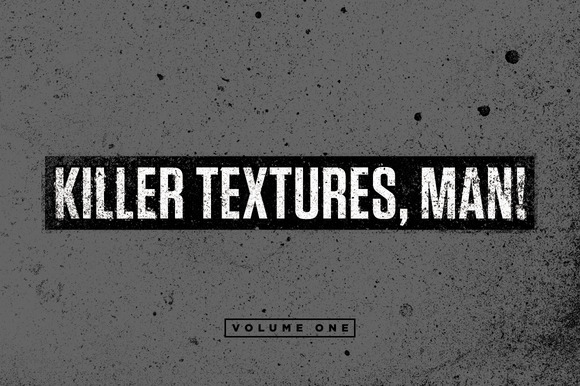The image features a dark gray background spattered with various black paint spots, creating a textured and multi-dimensional appearance. The black spots are of varying sizes, with some being larger and more prominent towards the upper part of the image, particularly in the upper right corner. In the center, there is a bold, elongated horizontal black rectangle. Inside this rectangle, thick white text that appears slightly smudged with black reads "KILLER TEXTURES, MAN!" in all capital letters, suggesting that this is a cover, possibly for a book or educational guide on achieving similar textures. At the bottom of the image, another black rectangle outlined in black lines contains smaller black text, also in all caps, that reads "VOLUME 1."